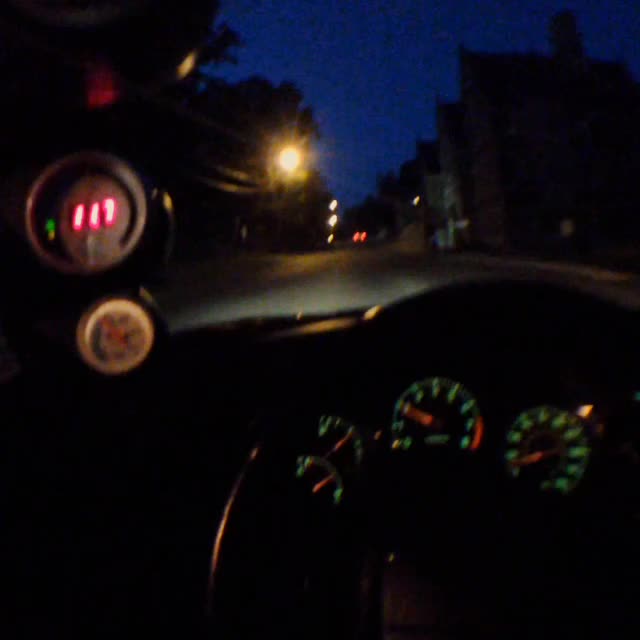This square photograph, taken from the driver's seat of a car at night or in the early hours of dawn or dusk, offers an intriguing view both inside and outside the vehicle. The dashboard is prominently lit up against the dim surroundings, showcasing circular displays with green backlighting, red pointers, and visible indicators for the RPM, MPH, and gas gauge. Above the windshield, a round device with an LCD screen displays the numbers "111" in red. Through the windshield, the scene outside is composed of a road lined with residential buildings on the right and trees and power lines on the left. The sky is a dark, navy blue, adding to the tranquil ambiance. In the distance, the red taillights of a car can be seen, and the road is illuminated by a series of streetlights emitting a soft yellow glow.